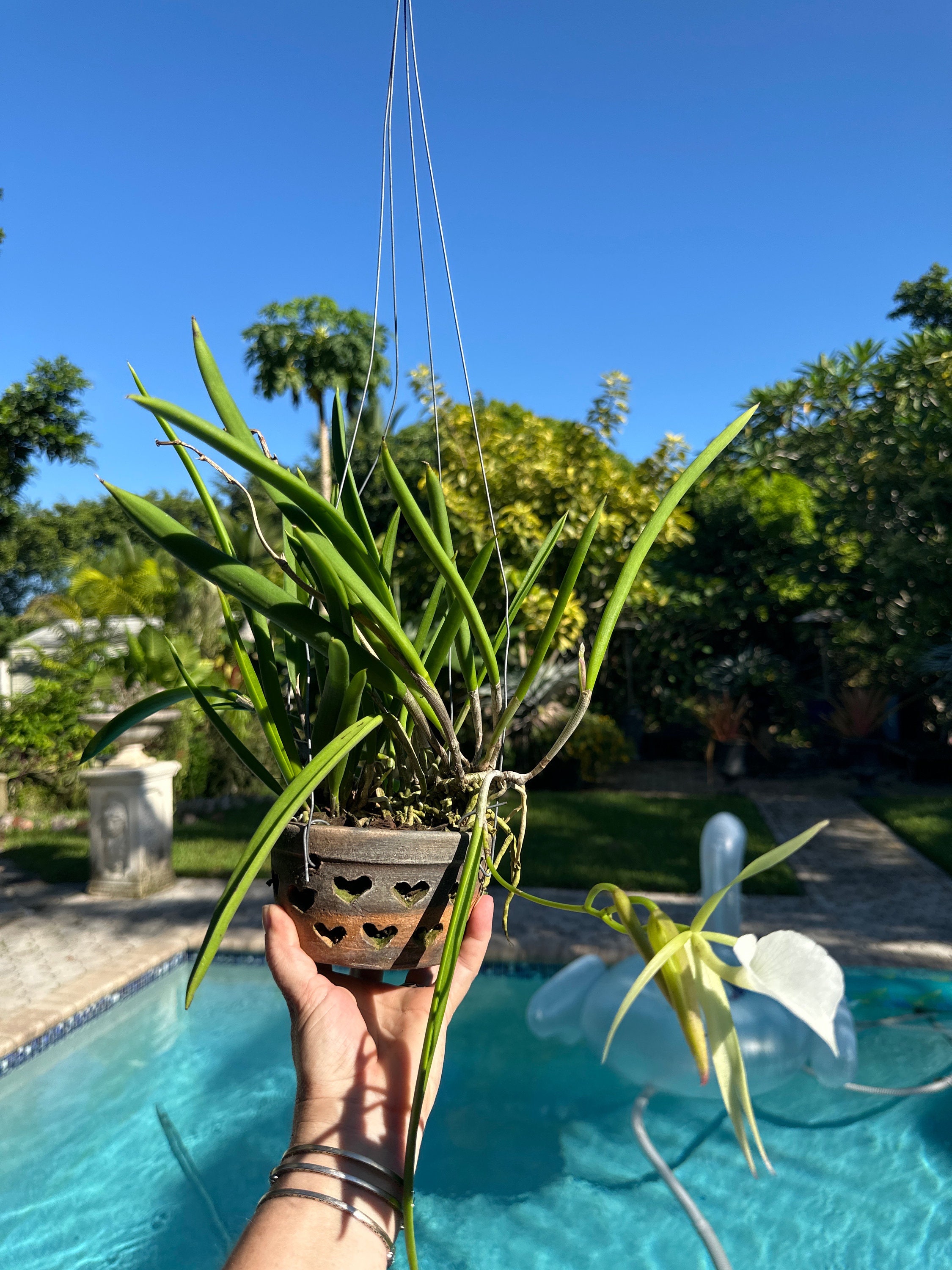In this outdoor photograph taken on a sunny day with a clear blue sky, we see an individual’s left hand extended over a pristine blue pool, holding a small potted plant. The hand, adorned with three silver bracelets, is palm-up, presenting a reddish-brown terracotta pot featuring heart-shaped cutouts. The pot contains a plant with long, slender, snake-like green leaves and a striking single white flower. Thin metal hanger wires extend from the top of the pot, suggesting it could be hung, although it is currently being held. The pool below has slight ripples, indicating a gentle breeze or recent disturbance, and is framed by beige and light gray flagstones. Surrounding the pool, there's a walkway leading under a canopy of lush, vibrant green trees, which add to the serene backyard setting. A clear, bright blue sky stretches above the scene, enhancing the tranquil atmosphere.